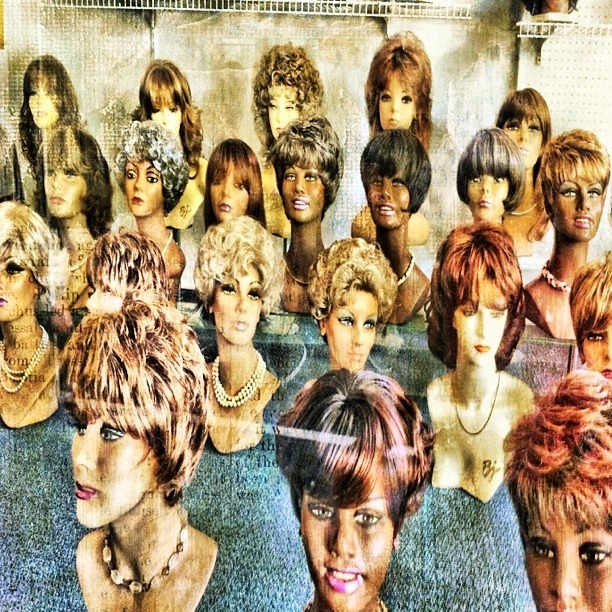This square-shaped photograph captures a striking collage of mannequin heads, each adorned with diverse and elaborate hairstyles. The mannequins, arranged on what appears to be a two-level cement table covered with a green cloth, display a wide array of wigs ranging from short bobs to longer styles that reach the shoulders. The wigs showcase a spectrum of colors, from blonde and red to black and gray, with some featuring curly and textured styles. Each mannequin head is intricately detailed, sporting full eye makeup and a variety of necklaces, though none have bodies. The heads are of different sizes and ethnicities, encompassing light-skinned and dark-skinned mannequins. A slight reflection on the lower left-hand side of the image suggests it might be photographed through glass or another protective covering. Additionally, one mannequin head prominently features the letters "BJ," possibly indicating the initials of the creator. The arrangement and details of the mannequins evoke the setting of a beauty or barber college, illustrating a grand display of hairstyling artistry.